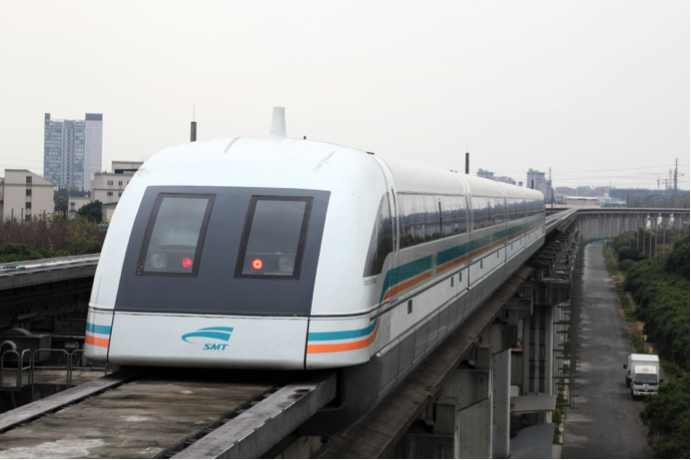The image depicts a white high-speed rail tram or monorail on an elevated track, appearing to curve to the right around the halfway point in the center view. The front of the tram features a row of dark grey vertical rectangular windows, with distinctive markings: the left window has a red line in the bottom right corner and the right window has an orangey-red line in the bottom left corner. Below the windows, there are two small rectangles forming a point and some blue text. The tram body also displays a dark teal stripe alongside an orange stripe running along its length. The track is above a road that features a big white van on the right, and adjacent to the road are a couple of trees and some green grass. The sky in the background is light grey, suggesting a foggy day, and on the left side, some tall buildings are visible against the skyline. Overall, the scene captures the tram either arriving at or departing from a station.